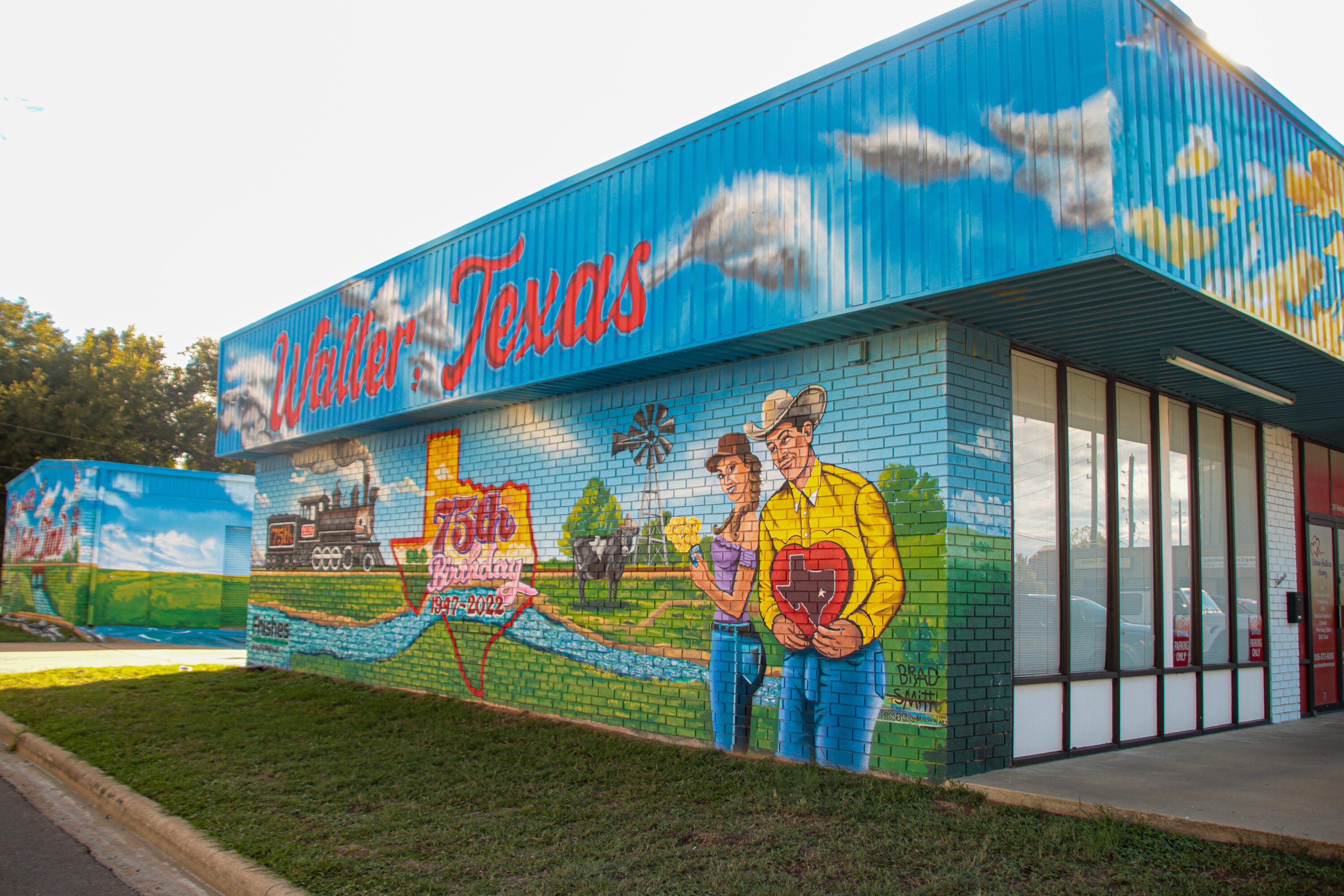The photograph depicts the exterior of a building, possibly the end unit of a strip mall or storage facility, adorned with a vibrant mural. The top of the building features a cloud-like design painted against a blue sky backdrop with red lettering that reads "Waller, Texas." Prominently displayed on the mural is the text "75th Birthday, 1947-2022," inscribed within the silhouette of the state of Texas. The mural is rich with details: a train is depicted driving through a town, a river winds its way through the scene, and green grass spans the bottom of the image. Additional elements include a cow, a western-style windmill, and a steer. There is a man wearing blue jeans, a cowboy hat, and a yellow western shirt holding a heart-shaped box of chocolates featuring the shape of Texas. Next to him stands a woman in blue jeans, a halter top purple shirt, a ponytail, and a brown hat; she is holding yellow daisies. An asphalt street with a concrete curb is visible at the bottom left-hand side of the image. In the background, another building with additional artwork can be seen, and a sign that says "Frisch's" is situated in the bottom left-hand corner of the main building. The composition suggests it is midday.